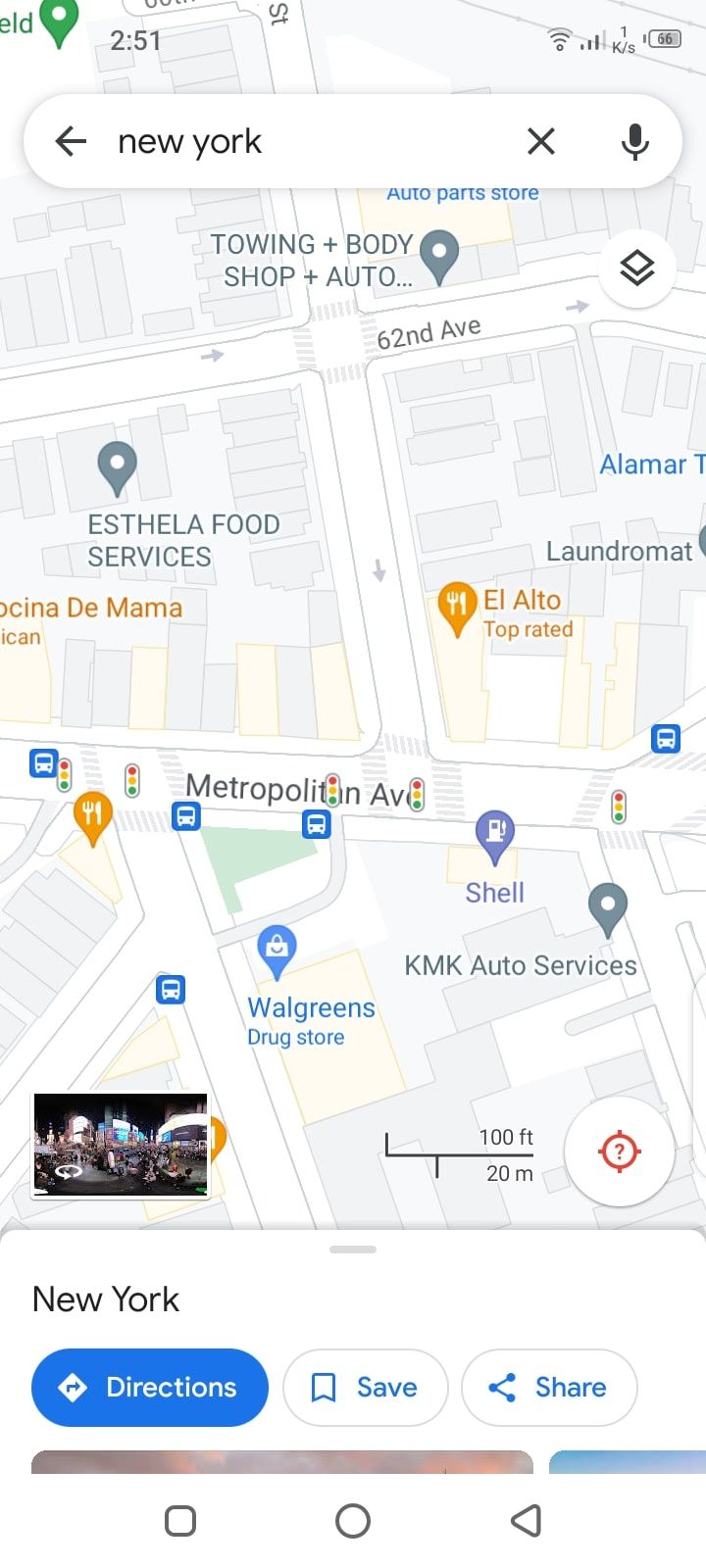This screenshot features a detailed map of a section in New York City, possibly viewed through either iOS Maps or Google Maps, as indicated by the slight differences in font. At the top of the screen, the current time is 2:51, with a Wi-Fi indicator showing moderate signal strength and a battery level at 66%. 

In the search bar at the top, "New York" is typed, accompanied by an 'X' and a microphone icon. Directly below the search bar, several locations are identified, including a Towing, Body, and Shop Auto situated on 62nd Avenue, and an Auto Parts Store positioned slightly above it.

On the map, various other landmarks and establishments are marked. To the left, Estella Food Services is listed, while to the right lies a network of roadways and buildings, likely commercial or residential. Key sites include a restaurant named El Alto, indicated by a fork and knife symbol, a laundromat, and a partially visible location called Olimar. Metropolitan Avenue is prominently featured with several traffic light icons, suggesting it is a busy thoroughfare.

Additional points of interest include a Walgreens drugstore, a nearby Shell Gas Station, and a map scale showing distances of 100 feet and 20 meters. At the bottom left corner of the map, there's a small image resembling Times Square, titled "New York," accompanied by options for directions, saving the location, and sharing it.